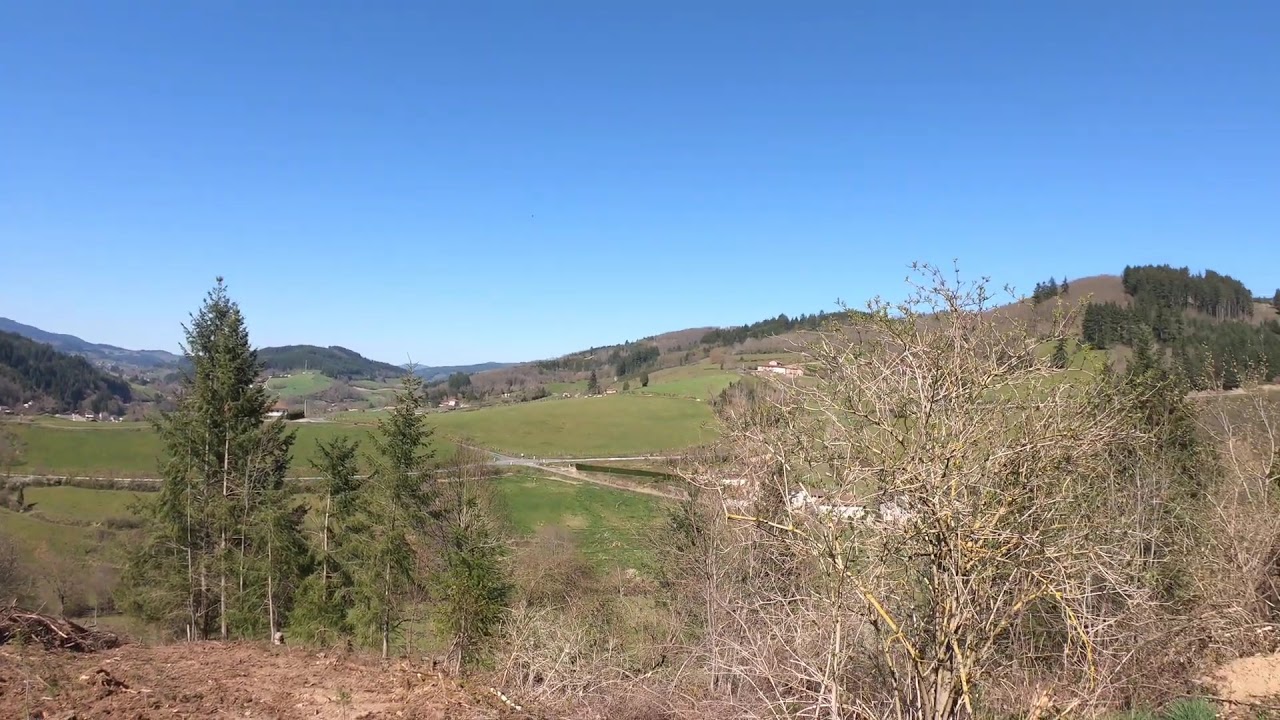This daytime photograph captures a serene, rural landscape from a vantage point on a hillside. In the foreground, the hill is dotted with a mix of green and dried, brown vegetation, including a few small pine trees on the left. The ground is a mix of bare dirt, scattered weeds, and dead bushes. As we move further into the view, the landscape transitions to lush, green grass fields intersected by multiple roads forming a grid. This area resembles a golf course, with manicured lawns and possibly a water feature running through the center, hinting at meticulously maintained grounds amidst the natural setting. In the middle distance, the terrain gives way to rolling hills adorned with sporadic dark green pine trees and patches of brown earth. Far beyond, the scene opens up to a picturesque mountain range, with its varying hues of green and brown, under a clear, cloudless blue sky. The sky's gradient from white near the horizon to a deeper blue at the top enhances the expansive, peaceful feel of the rural environment.